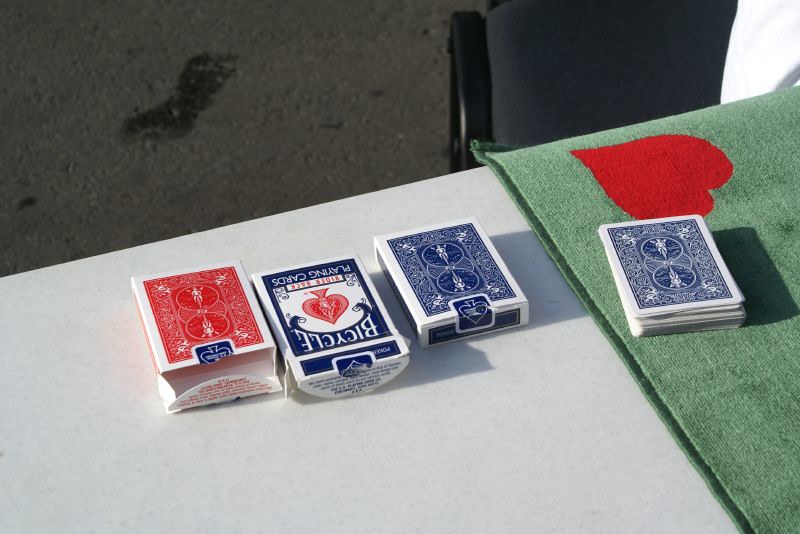The image captures a scene on a pristine white table surface adorned with various playing cards and decor. Prominently featured are three distinct boxes of playing cards. The first box, predominantly red with a card design, lies open with its back facing upwards. The second box, shown from the front, displays the iconic "Bicycle" branding along with a spade symbol and the words "Rider Pack Playing Cards." This box is also open. The third box, with a blue design typical of playing cards, remains sealed, evidenced by the intact sticker seal.

Amidst these boxes, a small green mat catches the eye, situated on the table and featuring a red heart in its center. Nearby, a neatly stacked pile of blue-backed playing cards rests face down. The background of the image includes a black railing or edge, possibly indicating the boundary of the table, with a darker area beneath it suggesting either a shadow or a dark carpet. The arrangement and varying states of the card boxes, coupled with the colorful decor, create a visually engaging tableau of casual gaming ambiance.